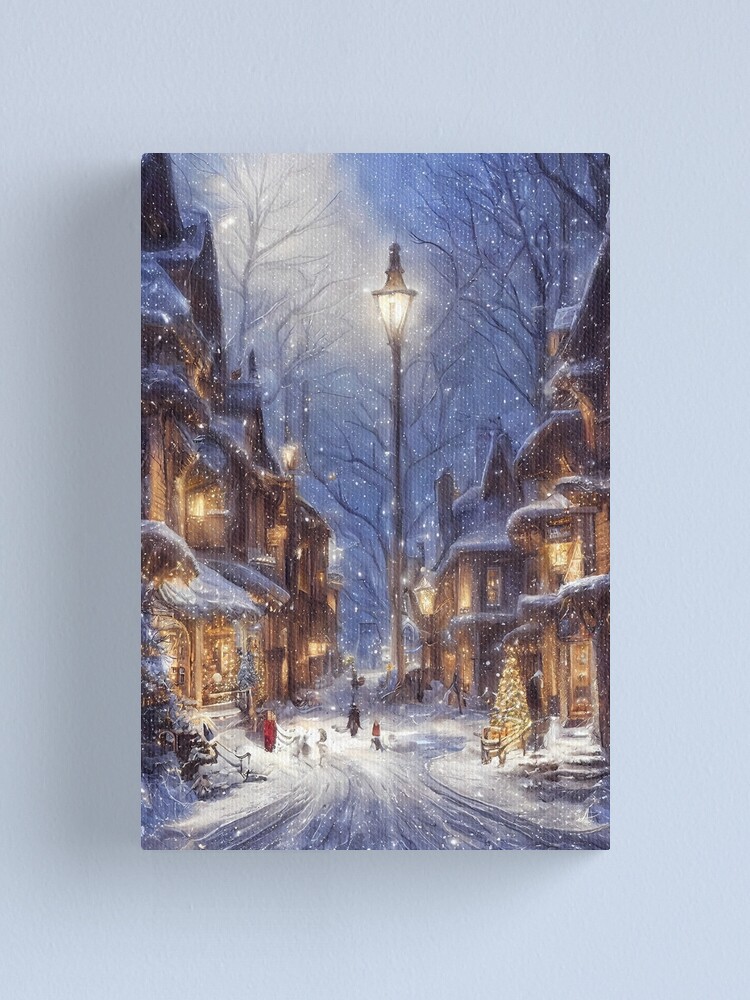This illustration captures a dreamy, wintry scene with meticulous detail. At the center of the painting stands a towering, black streetlamp that emits a warm, yellow glow, casting a comforting light over the surroundings. The sky is a soft blue, adorned with a gentle snowfall that blankets the landscape. Flanking the dark asphalt road, covered in snow and ice, are two- and three-story homes with brown exteriors and snow-covered rooftops, their windows glowing warmly from within. Tall, thin, leafless trees stretch their spindly branches toward the sky, adorning the scene and emphasizing the season. 

On the right side of the street, a well-lit Christmas tree stands resplendent with ornamental yellow lights, mirroring the festive decorations that glitter on the trees lining the road. People dressed in winter clothing—reds, blacks, and more reds—walk amidst the scene, adding life and vibrancy to the postcard-perfect setting. Steps lead up to the front door of the house immediately on the right, inviting one into the warmth. The entire scene evokes the serene and cozy spirit of Christmas, with every detail contributing to a picturesque winter wonderland.